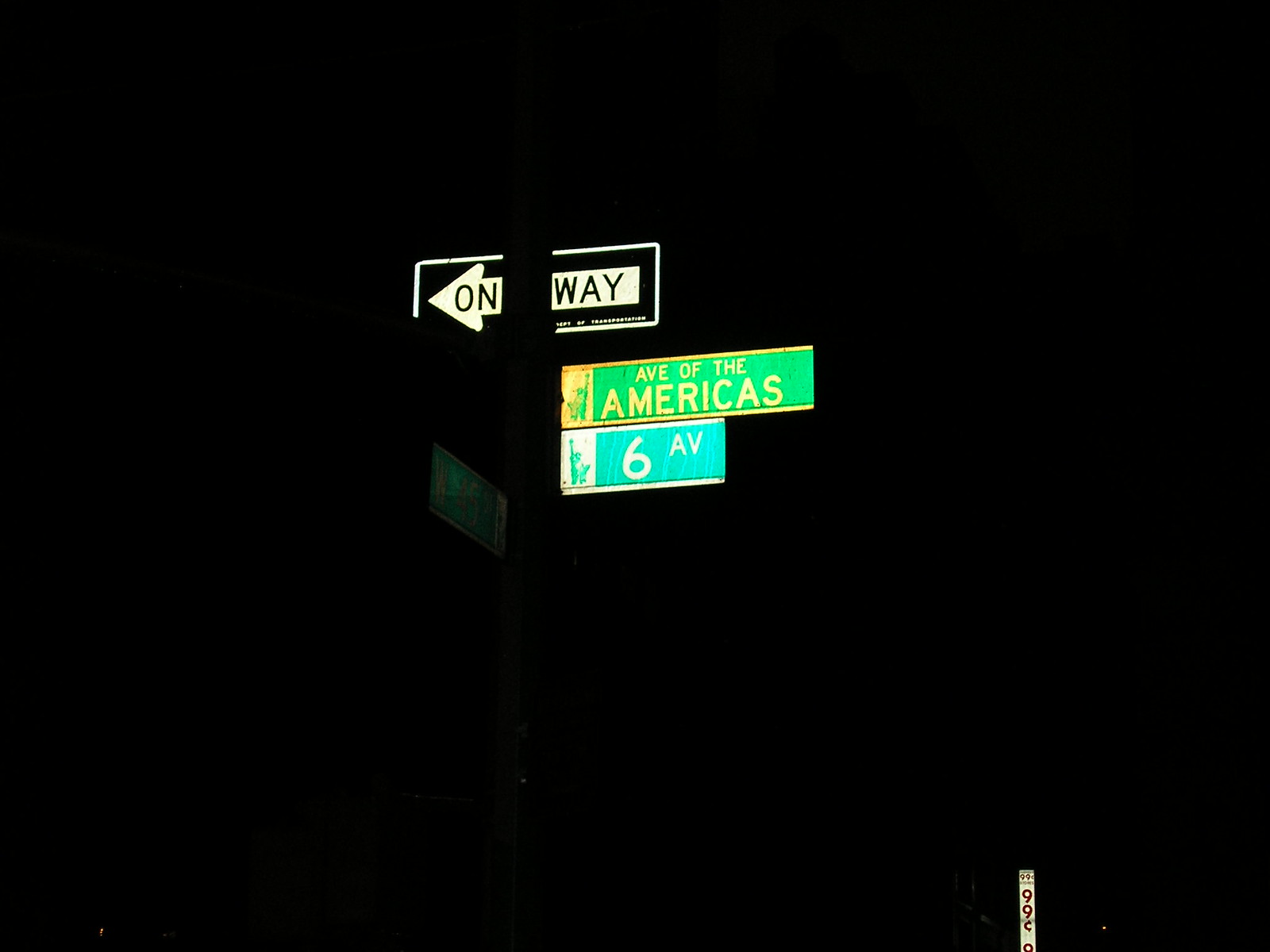A nighttime photograph captures a nearly pitch-black scene, offering a fleeting glimpse into a city intersection. Dominating the center, a one-way street sign, its arrow pointing left, is partially obscured, leaving only "ON WAY" visible. Just below it, a green street sign displays "AVE OF THE AMERICAS," accompanied by a light blue sign that reads "6AV." Nearby, an indiscernible sign tilts sideways, adding to the cryptic ambiance of the image. In the lower right-hand corner, a small, brightly-lit sign advertises "99¢," providing a stark contrast to the overall darkness enveloping the scene.